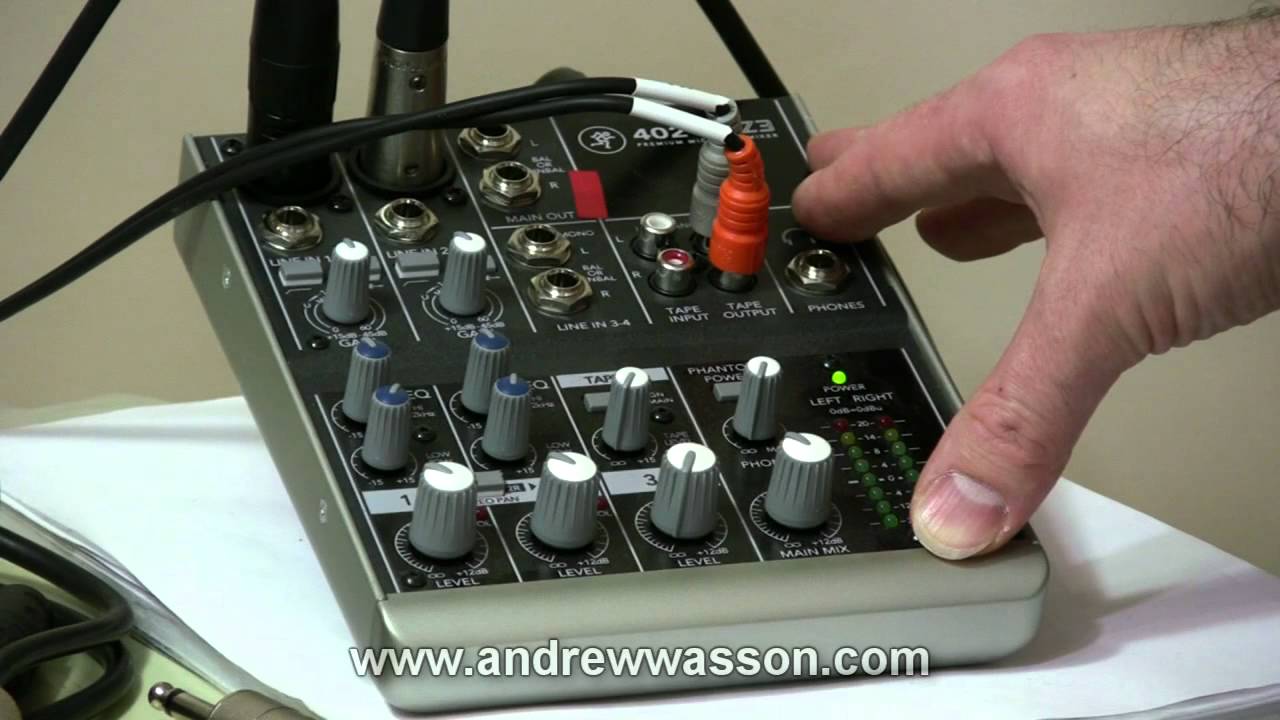The image features a compact audio mixing device with a grey and black color scheme, resting on a table scattered with papers. The device belongs to someone associated with www.andrewwasson.com, as indicated by the text at the bottom. A man's right hand is depicted adjusting controls on the mixer, suggesting he is an audio engineer. The mixer includes a variety of buttons and dials: 

- Main out
- Tape input/output with red and grey cables plugged into the output
- Phones
- Power
- Left and right buttons with green decibel indicator lights
- Main mix
- Three level buttons at the bottom
- Four dials with blue tops 
- Two additional dials above the blue ones
- Several unoccupied input jacks

Notably, the mixer appears branded with a series designation, possibly "402Z3," and features colorful knobs to adjust frequencies and volume levels.